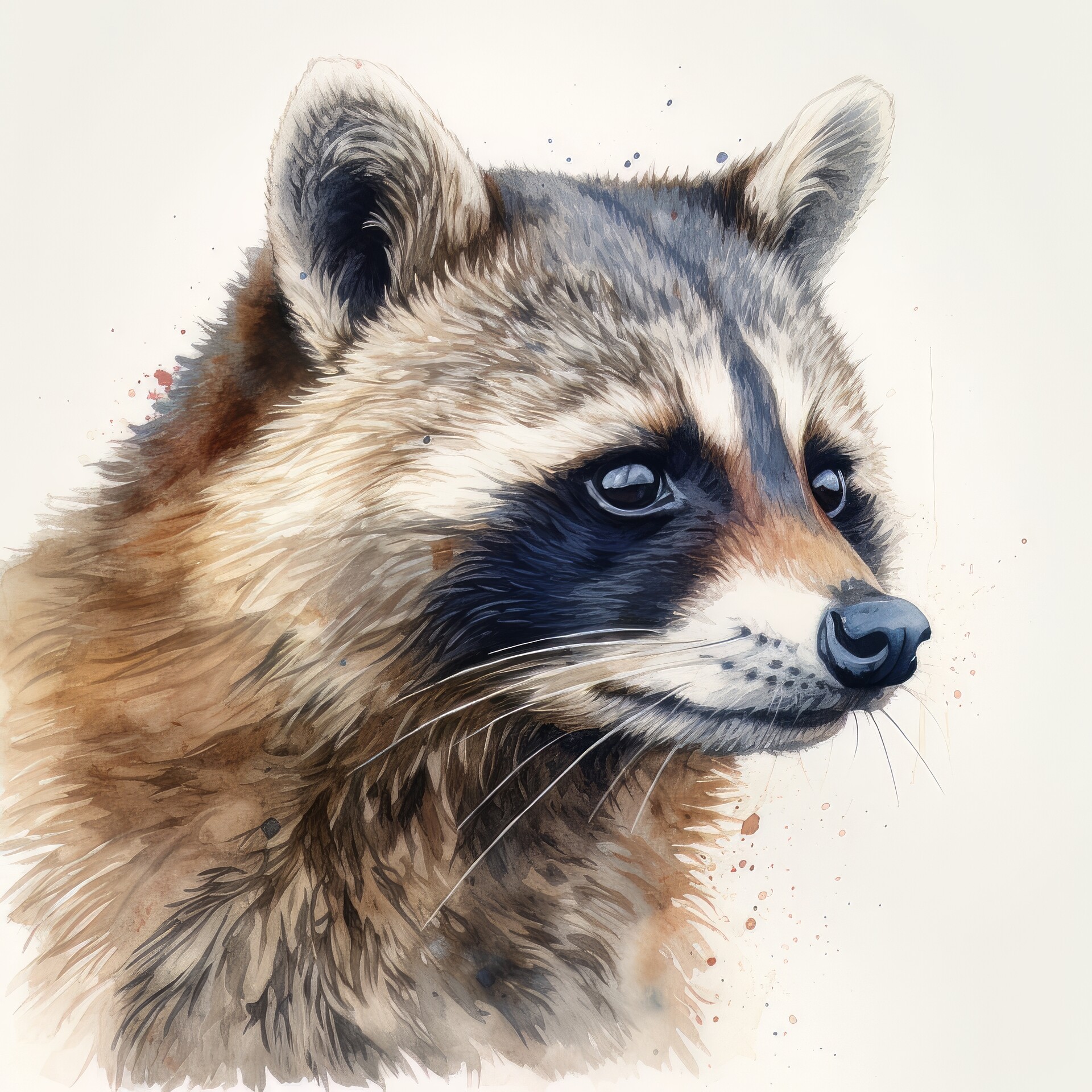This image is a digitally created, semi-realistic drawing of a raccoon's head set against a beige or off-white background. The raccoon is depicted in a three-fourths profile, looking to the right with a blank stare. The fur is colored in shades of brown and white, with distinct dark black eyes that have a noticeable reflection. The raccoon's white ears have black centers, and a prominent black stripe runs from the top of the head down to the top of the nose. The area around the eyes is also black, which contrasts with the brown top of the nose and the black nose itself, which is outlined in white fur. White whiskers sprout from the raccoon's muzzle, and the fur extending down the neck incorporates both brown and black hues. The overall style is convincingly painterly, with the digital technique giving the appearance of a traditional painting.